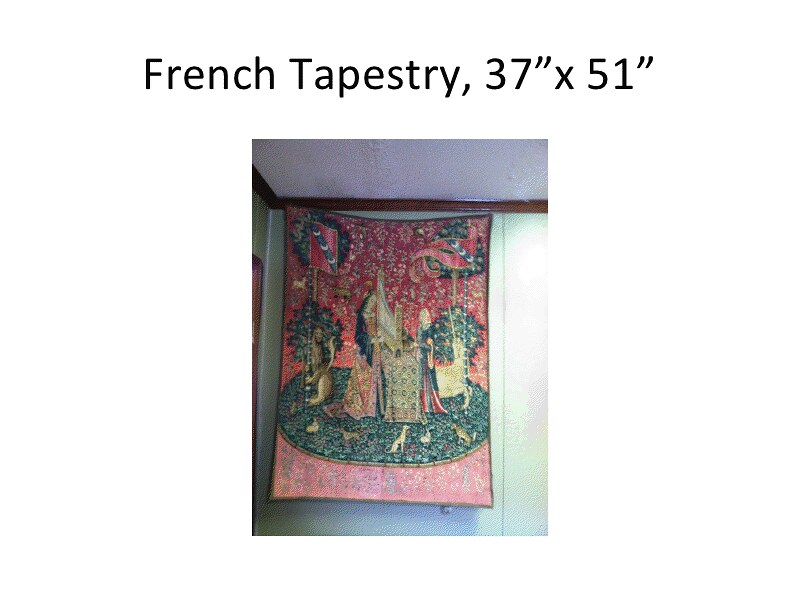In this photograph, we see a detailed French tapestry measuring 37 inches by 51 inches, prominently labeled at the top. The tapestry features a vibrant red background that transitions from a darker hue at the top to a lighter hue at the bottom. At the top right, there is a decorative element resembling a boat anchor adorned with various objects. The top left corner features a Christmas wreath, partially obscured by a banner held by a lion-like creature. This creature supports a pole topped with a banner that has red and white rings.

Central to the scene are two women positioned on a green circular ground that looks like a carpet. One woman appears to be engaged in a craft, possibly knitting or operating a threading machine, while the other woman stands nearby, perhaps holding a harp. Surrounding these figures are various plants and greenery, including a tree with a bushy base and a slender trunk.

The background reveals additional details: a white paneled wall with brown trim at the top, and a white ceiling that looks recently repaired. To the right of the crafting woman, there is what appears to be a bassinet with a shade above it. A couple of small bushes and two dogs are also present on the green carpet, adding to the intricate and rich details of the tapestry scene.